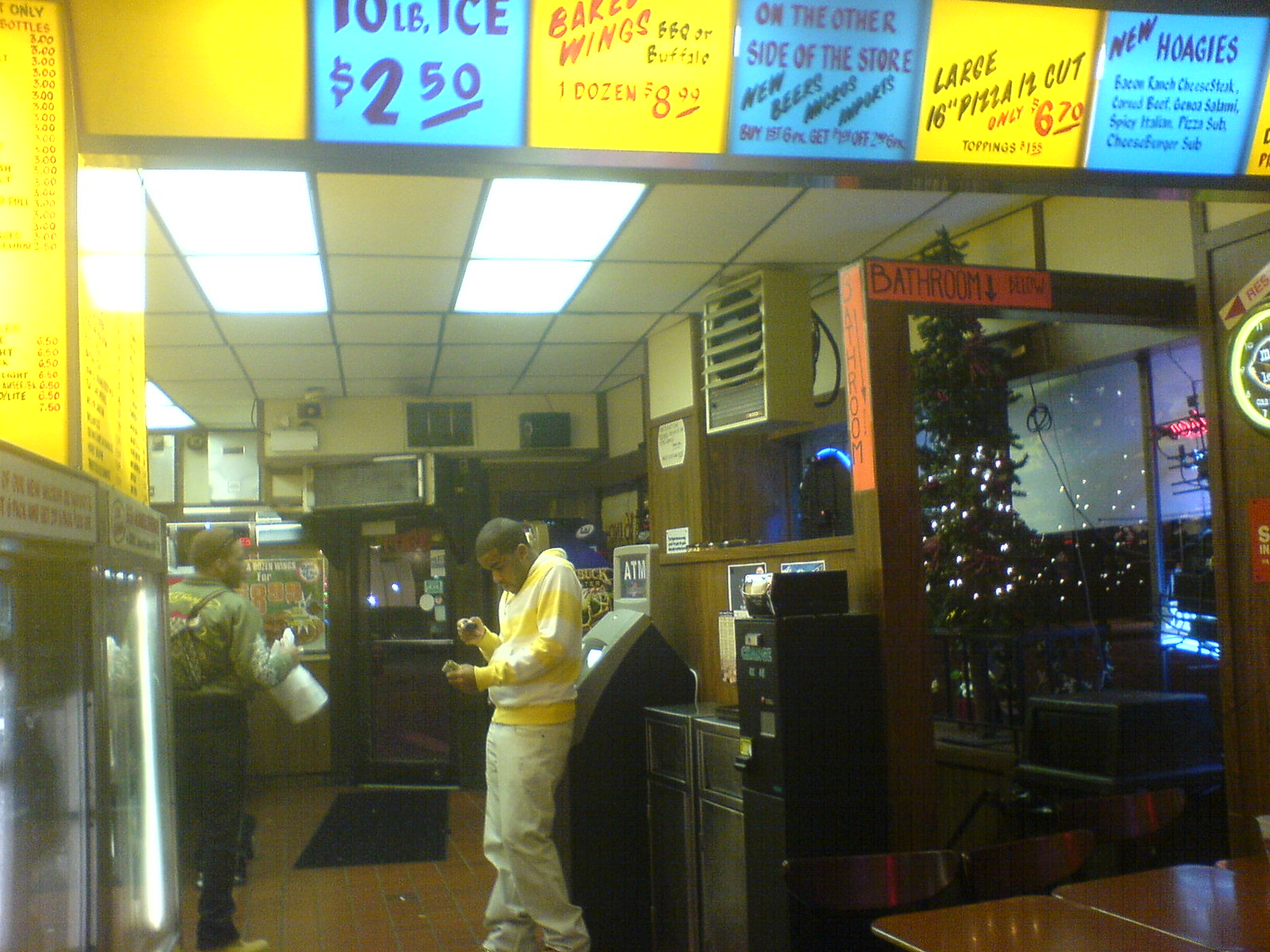The photograph captures the interior of a convenience store with fluorescent lighting inset into yellow ceiling panels outlined in black. The walls are a tan color complemented by wood accents at the lower sections. A prominent banner runs across the top of the image, featuring yellow and light blue panels that advertise various items such as "10 pounds of ice - $2.50", "baked wings - 1 dozen for $8.99", "large 16-inch pizza - $6.70", "new beers and imports", and "hoagies".

In the foreground, two customers are present. A black male with very short hair, dressed in a yellow and white striped long-sleeve shirt and white pants, leans against an ATM, absorbed in his phone. To his left is another man wearing a green jacket with a design on the back, holding an indistinct white object, possibly paper towels.

On the right side of the image, there's a door labeled "bathroom" with an orange banner and an arrow pointing downward. Above the door, a wooden frame can be seen, and nearby, there is some indoor greenery adorned with Christmas lights, hinting at a wintertime setting. The store’s floor is brown, and a wooden table is positioned in the lower right corner. Ventilation systems run along the upper and right edges of the image, and behind the man in the yellow shirt, an ATM and additional black machine are visible. Lastly, a black rug lies in front of a doorway further into the store.